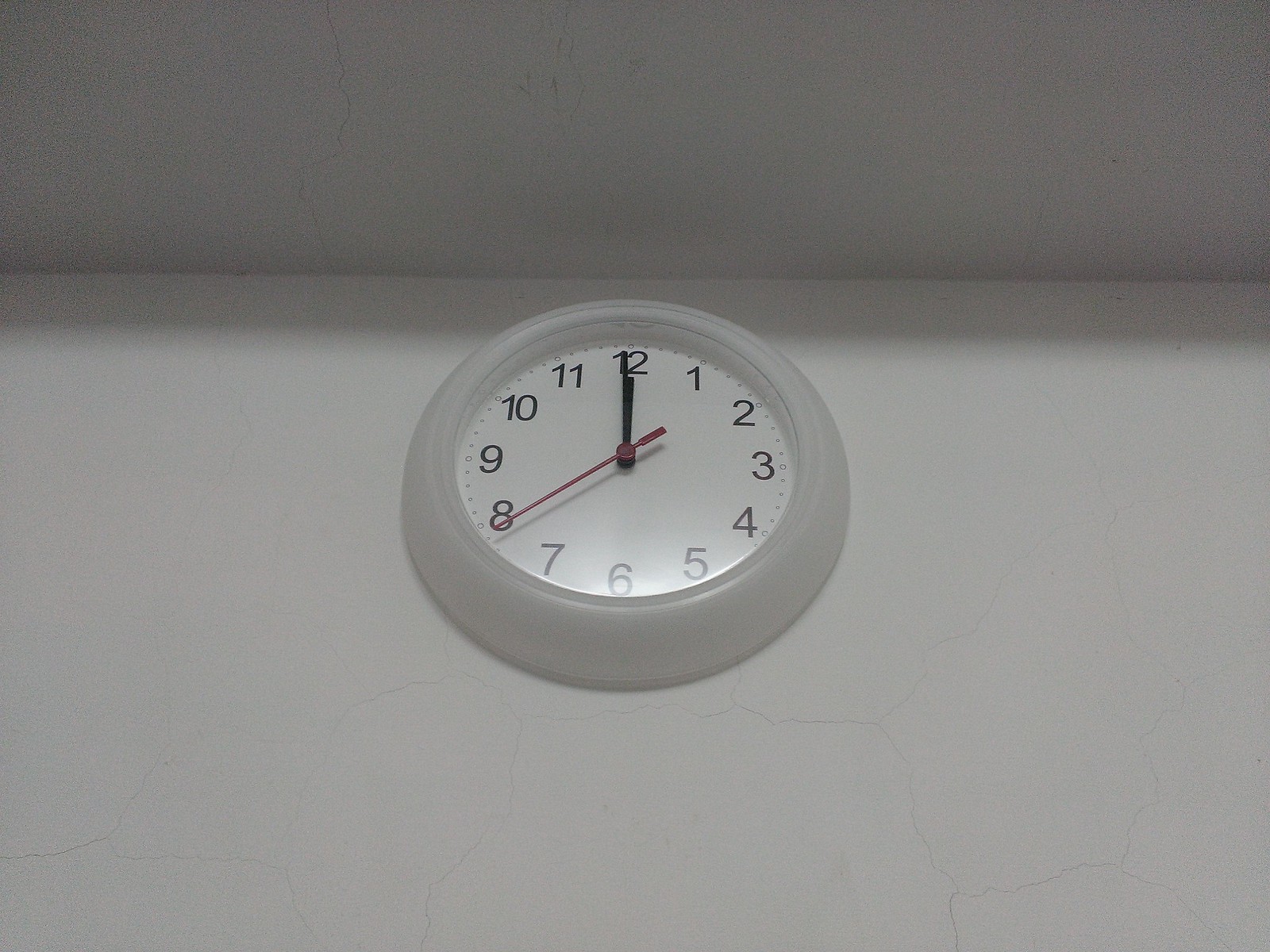This photograph captures a minimalist clock mounted high on a pristine white wall, nearly brushing the crisp, white ceiling. The clock's design is strikingly simple yet elegant, featuring a white frame and a matching white face adorned with bold, black numerals and minute notches. The clock is equipped with three hands: the hour and minute hands, which are both sleek and black, align precisely at the 12 o'clock position, while the second hand, a contrasting vivid red, points to the 8-second mark. Subtle shadows cast by the ceiling add a touch of depth and dimension to the top of the wall, highlighting the clock's placement and sparking visual interest in an otherwise stark space.